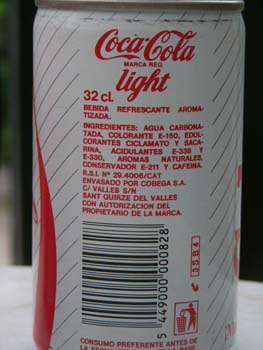This is a close-up, color photograph of a can of Coca-Cola Light placed on a white marble countertop with light gray streaks. The Coca-Cola logo, written in iconic red cursive text, prominently displays the elongated loop of the "C." Beneath the logo, "Light" and "32CL" are also written in cursive text. The can's background is white, indicating it’s a diet variant. In Spanish, the ingredients list begins with "aqua." Directly below the ingredients list is a barcode with the sequence "5449-000-000-828." Adjacent to the barcode is a small red-bordered rectangle featuring the number "3584" in red. Additionally, there is an icon depicting a person tossing the can into a trash receptacle, suggesting proper disposal. The photograph primarily focuses on the can against a dark, indeterminate background.